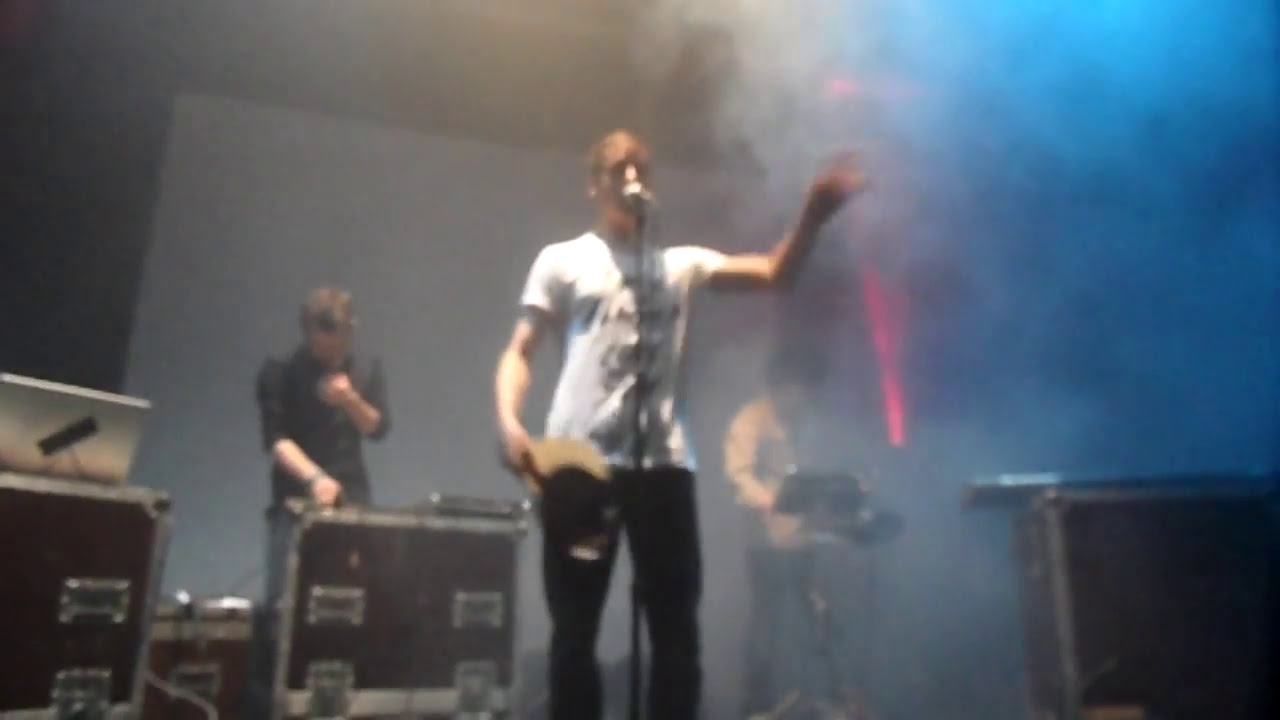The photograph captures an indoor concert scene, featuring three musicians performing on a smoky stage. The central figure is a white man wearing a white t-shirt with black lettering and black pants, passionately singing into a microphone. His left hand is raised, gesturing towards the blue and grey smoke that fills the room, with a concentration of blue smoke and a red laser light visible on the right side. Behind him to the left, another white man in a black shirt stands at a brown wooden contraption with a silver exterior, possibly a DJ station. To the central figure's right, a third musician, dressed in a long-sleeve yellow or orange collared shirt and dark pants, is faintly visible through the smoke, seemingly at a drum set. The image is blurry and appears to have been taken from a low angle near the ground, with the dense smoke and low lighting adding to the hazy, atmospheric feel of the concert setting.